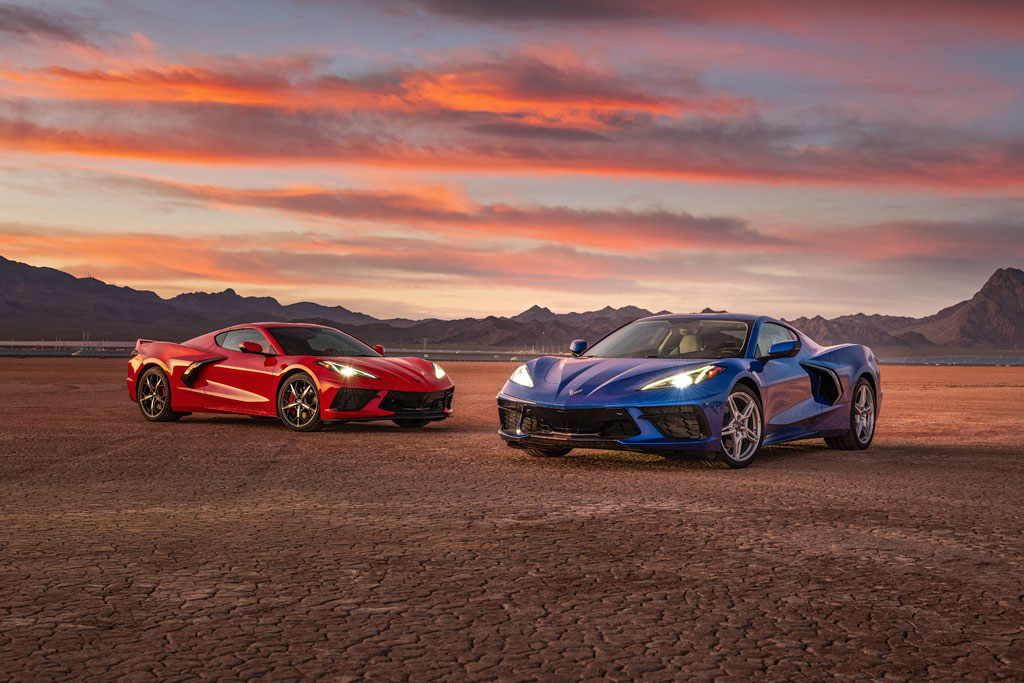This photograph features two modern mid-engine Corvette sports cars set against a picturesque desert landscape. The car on the right is blue, while the one on the left is red; both vehicles have their angular headlights turned on, casting a glow on the hard-packed and slightly cracked sandy terrain. Positioned in a three-quarters view, the blue Corvette appears to face the left side of the image, while the red Corvette, just slightly set back, faces the right side. Notably, both cars feature black air intakes located behind their doors and have their engines mounted in the rear, just ahead of the rear wheels. The backdrop showcases a rugged mountain range under a sky painted with hues of orange, pink, and blue, indicating the sun has recently set, although the sun itself is not visible. The atmosphere reflects a serene yet dramatic twilight, with clouds tinged with shades of pink, white, and gray, adding depth to the scene.